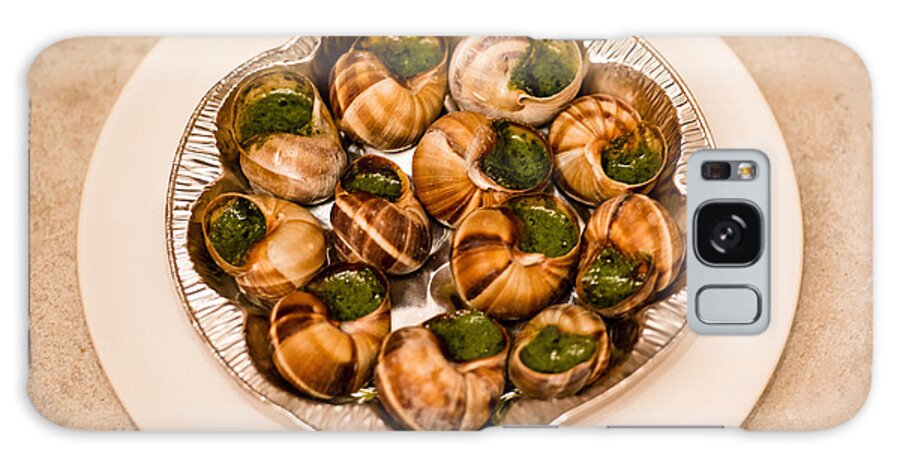This close-up image showcases a plate of food in a detailed and intricate manner. At the center is a white ceramic plate, topped with a smaller aluminum foil plate. The foil plate contains approximately a dozen large, dark orange snail shells arranged in a circular pattern, each shell stuffed with a vivid green filling. Off to the right side of the image, a silver or gray camera (which might be a phone) is partially visible. The camera, oriented horizontally, features a lens and possibly a flash, and appears significantly smaller relative to the dish it's placed beside. The table beneath the plate appears to be of a matching eggshell white color, further emphasizing the clean and bright aesthetic of the scene.